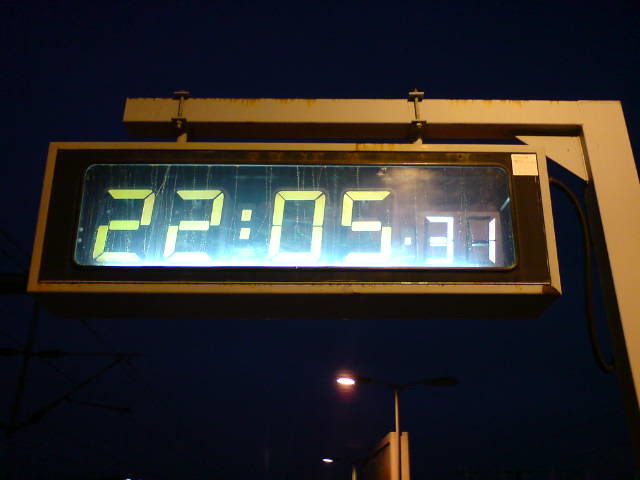A digital race timer is prominently displayed in this nighttime or early morning scene, suspended from a gold-brown metal arm that forms a right angle. The LED display, glowing brightly in greenish-yellow, reads "22:05.31." The timer is likely used for an ultra-marathon or Ironman race, given its outdoor setting. The sky is an intense dark blue, indicative of either night or the early hours before dawn. A distant light source illuminates part of the background, adding depth to the image and highlighting the sense of anticipation and quiet typical of pre-race or late-night moments.